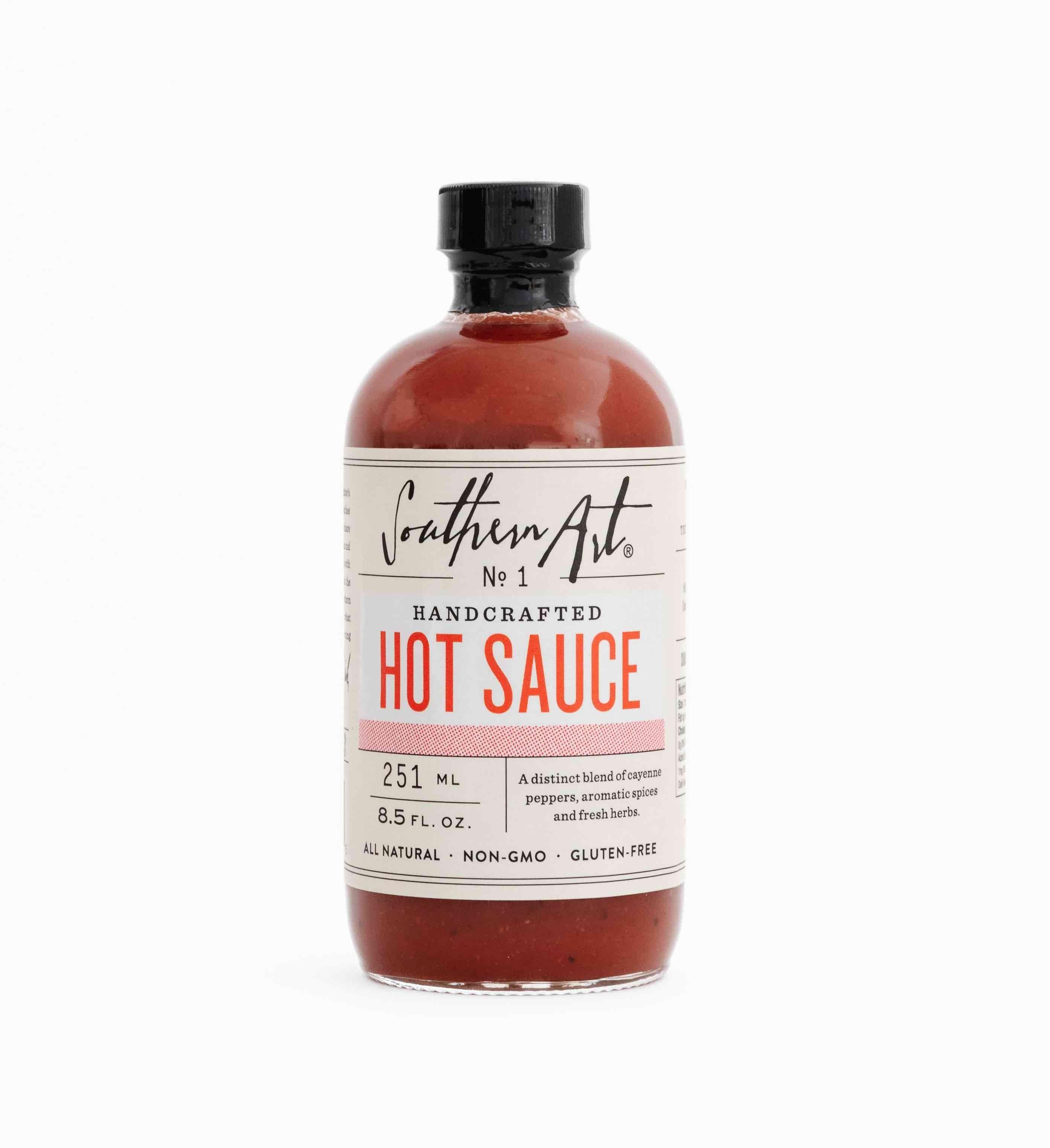This image features a square-shaped photo, 6 inches by 6 inches, with a very light gray background, emphasizing the central object—a bottle of hot sauce. The glass bottle, approximately 3-4 inches high, widens from a 1-inch base to about 1.5 inches at its broadest point, and tapers to a thin, narrow neck covered in black paper, capped with a twist top. The label on the bottle is a light tan or ivory color adorned with black cursive text reading "Southern Art," followed by "Number One Handcrafted," and the words "Hot Sauce" in bold red or bright orange print. The label indicates that it’s an 8.5 fluid ounce (251 milliliters) bottle, containing a distinct blend of cayenne peppers, aromatic spices, and fresh herbs. The hot sauce inside is a dark reddish-orange color. Notably, the product is marketed as all-natural, non-GMO, and gluten-free. The bottle appears transparent, showcasing the sauce within. The simplistic gray background focuses attention on the bottle, suggesting the image is likely used for online product advertising.